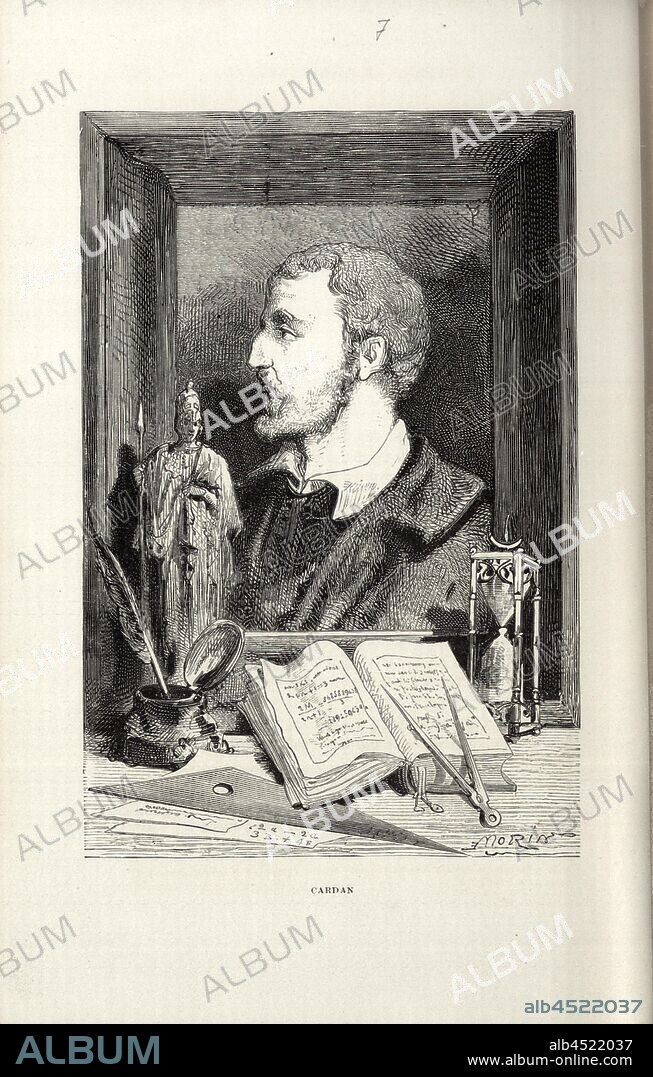The photograph features an intricately detailed still life on an old English tabletop. Central to the composition is a black and white pencil sketch of a noble-looking man, viewed in left profile, housed in a wooden picture frame. He has curly hair, a strong nose, sparse facial hair, and is dressed in a white collared shirt with a jacket. The grayscale illustration hints at his scholarly or philosophical stature.

Surrounding the portrait, the tabletop hosts an array of objects: a meticulously placed protractor rests atop an open book, a square for measurements sits nearby, and an hourglass counts time beside them. A tall statue draped in robes, donning a hat and holding a sword, stands upright, adding to the scholarly ambiance. Also present are a feather quill and an inkpot, indicative of classic writing practices.

Beneath the frame, the name "Cardan" is inscribed, and at the photograph's bottom, the artist's signature "Morin" can be discerned. The image is watermarked repeatedly with the word "album" to prevent unauthorized copying, and the web address www.album-online.com along with identification code ALB 4522037 is printed in lighter black at the bottom, providing a distinct marker for this detailed and evocative still life.